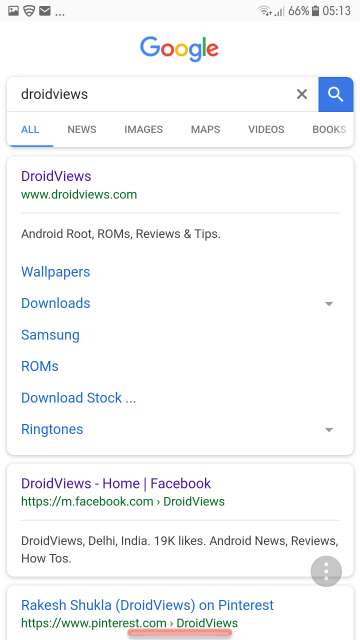This image appears to be a screenshot taken from a smartphone displaying a Google search results page. At the top of the screen, the phone displays its status bar, which includes various icons and notifications: Wi-Fi signal strength, cellular signal bars, a battery level of 66%, and the current time of 5:13 PM. Below the status bar, the Google logo is displayed in its classic rainbow colors, and the search query entered is "droid views."

The search results interface shows that the 'All' tab is selected in blue, while other tabs like News, Images, Maps, Videos, and Books remain in black. The first search result is highlighted in purple with the website "www.droidviews.com" shown in green beneath it, followed by a description in black text stating, "Android root ROMs reviews and tips." Below this description, there are links for "Wallpapers," "Downloads," "Samsung ROMs," "Download Stock," and "Ringtones," with "Ringtones" highlighted in blue.

Further down, there is another search result in a purple rectangular box indicating "Droid Views - Home/Facebook," with a link to "facebook.com/droidviews." This result includes an additional description stating "Droid Views - Delia India, 19k likes - Android news, reviews, how-to's," followed by a link to Pinterest in green.

The detailed nature of the screenshot captures a well-organized layout of Google search results, effectively showing the various links and information related to "Droid Views."